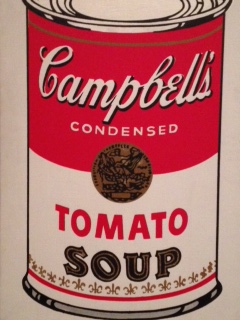This image is a stylized, vertically aligned illustration of a can of Campbell's Condensed Tomato Soup, reminiscent of Andy Warhol's iconic pop art. The can is prominently displayed against a white background. The top of the can is adorned with the cursive "Campbell's" logo in white, set against a rich red background, followed by the word "Condensed" in a block font. Below this, a central golden seal, though not entirely legible, adds an element of vintage design. The lower half of the can is white, bearing the bold red lettering "Tomato" and "Soup" in an old-fashioned black font. Subtle details, such as a fleur-de-lis gold pattern and a slight red line, further embellish the bottom of the can, providing a touch of classic elegance.